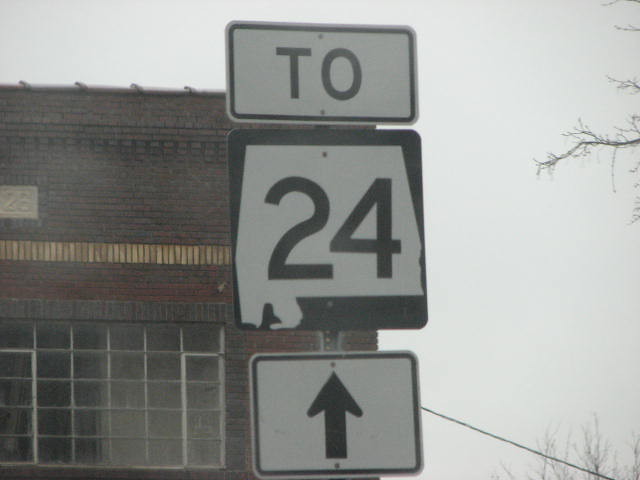This photograph captures a vertical road sign featuring three distinct signs against an urban backdrop. The top sign has a white background with a black outline and displays the text "TO" in black font. Below it, the middle sign has a black background and showcases a white silhouette of a state, potentially Nevada, although the exact state isn't clearly identifiable, along with the number "24" in black. The bottom sign is white with a black outline and features a black arrow pointing upward. Behind the road sign stands a red brick building with a large multi-paned window, suggesting an older architectural style. To the right, the scene includes some bare trees devoid of leaves, indicating a fall or winter setting. The sky above appears overcast, with a dull white or gray hue.